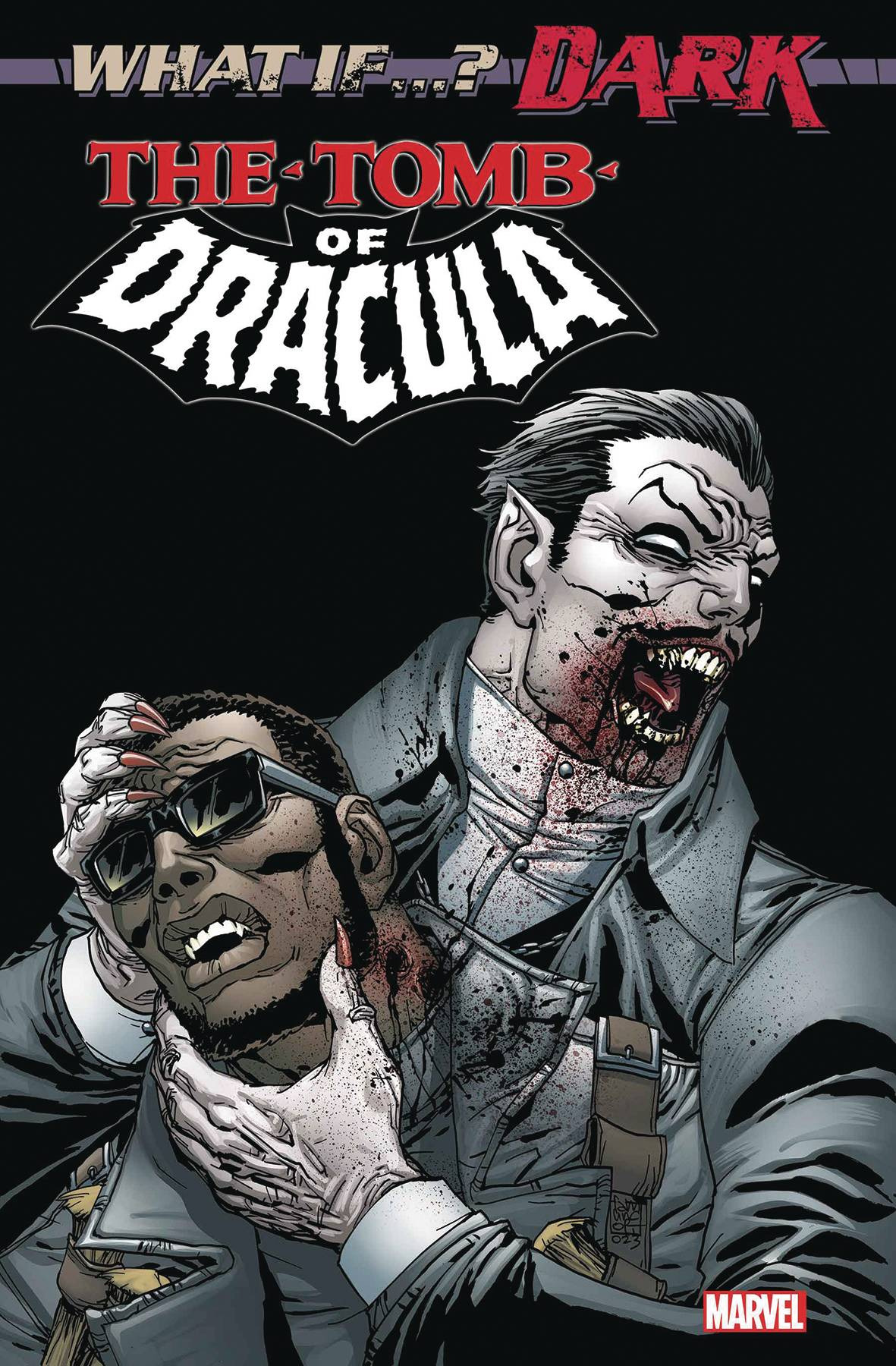The comic book cover for "What If...Dark: The Tomb of Dracula" features a chilling and violent scene under the iconic Marvel banner, located in white text with a red border at the bottom right corner. Dominating the central illustration is a fearsome vampire, garbed in a high-collared white shirt and dark jacket, clutching the head of his recent victim with both hands adorned in red fingernail polish. The vampire, identified by some as Dracula, has his mouth smeared with blood, indicating a recent bite on the throat of the victim—whose neck bears two red puncture wounds. The victim, believed to be Blade, a famed vampire hunter often portrayed by Wesley Snipes in films, appears powerless beneath the vampire’s grasp. Above this gruesome tableau, the comic title is prominently displayed: "What If...Dark" in brown and red text, with "The Tomb" and "Of Dracula" creatively embedded within a black bat outline.